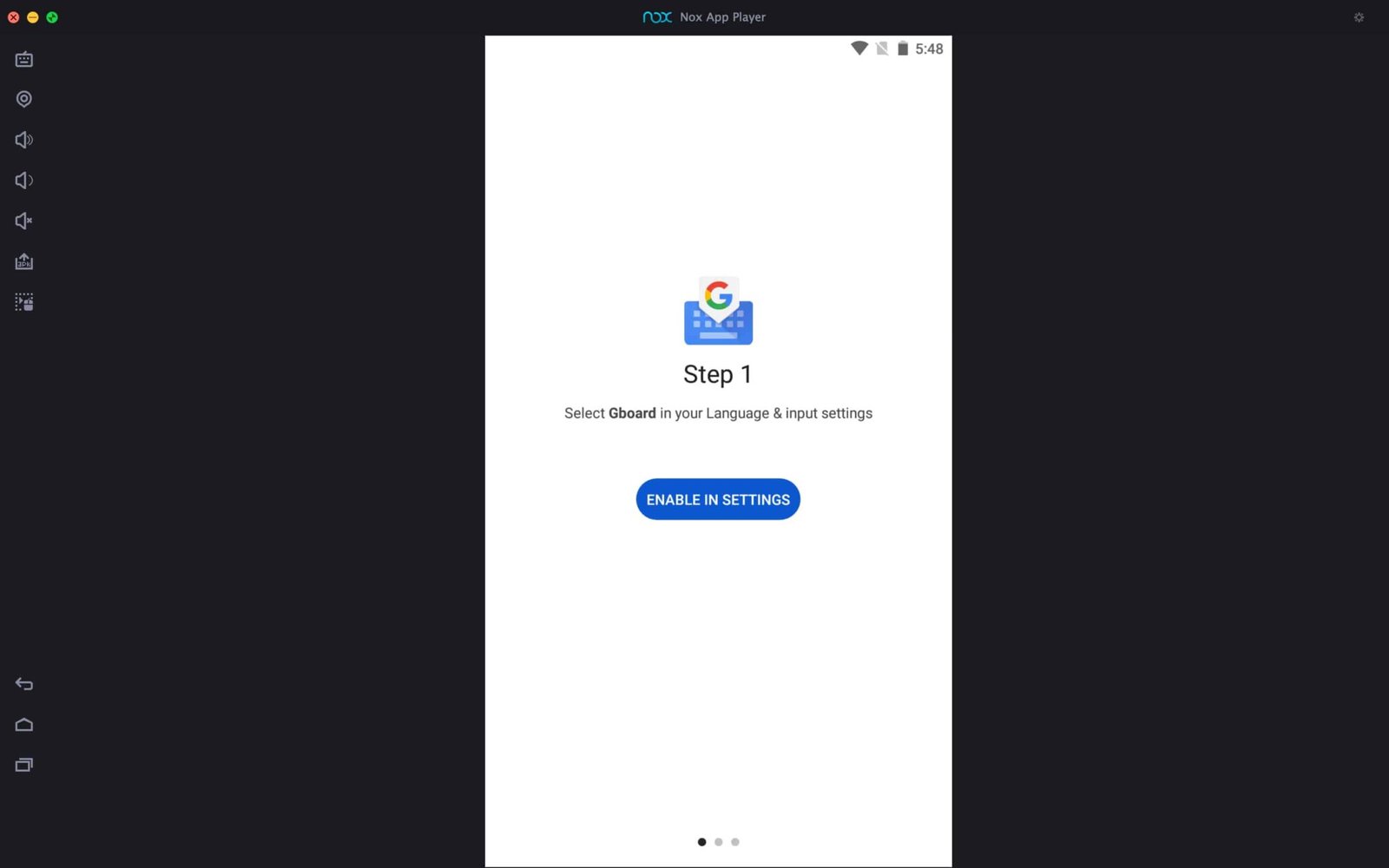This is a screenshot of a Knox App Player setup screen with a predominantly black background. At the center of the screen is a tall, vertical white rectangle. In the far upper left corner, three circles appear in a sequence: red, orange, and green. Below these circles is a series of white-outlined icons. The first icon resembles a radio, followed by a circle within a circle. The next three icons depict a sound speaker projecting sound, a smaller sound speaker, and a sound speaker with an 'X' behind it, symbolizing mute.

At the top of the screen, in blue text, it says "Knox," followed by white text reading "Knox App Player." Inside the white rectangle, in the upper right corner, there is a Wi-Fi signal icon next to a square with a cross through it, a battery indicator, and black text displaying "5:48." 

Centrally located within the rectangle is a blue keyboard icon adorned with the Google emblem, which features the letter 'G' in red, yellow, green, and blue. Below this icon, in black text, it says "Step 1." The text instructs users to "Select Gboard in your language and input settings." Finally, at the bottom of the white rectangle, there is an oblong blue oval button with white text reading "Enable in Settings."